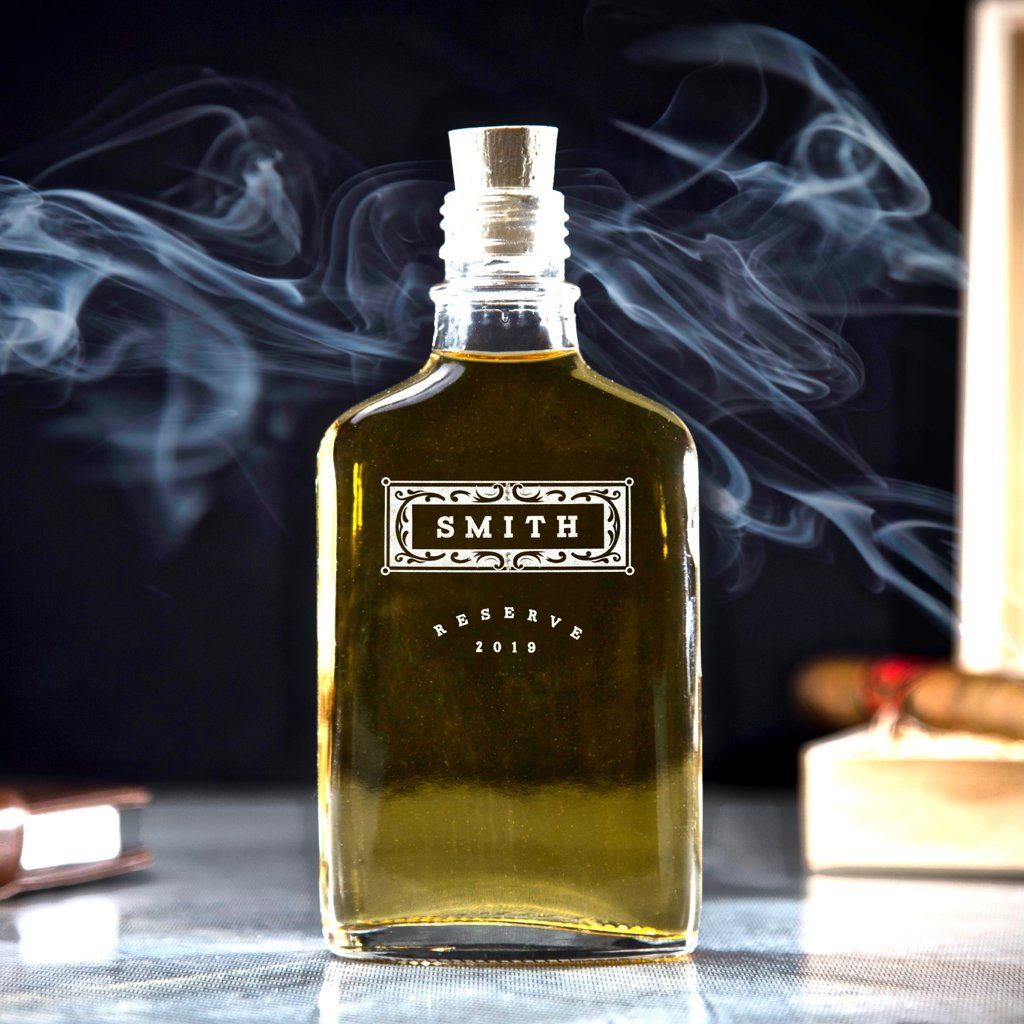This evocative photograph, likely an advertisement, features a bottle of fine liquor set against a moody, dark background. Central to the composition is a rectangular, pint-sized bottle filled with an amber liquid that nearly reaches the bottle's neck. The bottle, adorned with a tan cork stopper, sits on what appears to be a reflective marble or granite surface. 

Prominently displayed on the bottle is a label that reads "Smith" within a florally adorned rectangle. Below this, the label also states "Reserve 2019", following a curved format. The liquid inside takes on a golden hue, influenced by the dark setting, giving it a rich, appealing glow.

In the background, slightly out of focus, there's a smoking cigar placed on an open cigar box to the right, its brown wrapper accented by a red band. Swirling gray smoke from the lit cigar enhances the atmosphere, trailing across the scene from right to left. On the left side, one can make out a copper-toned object and a book, tying into the overall theme of sophisticated leisure—inviting the viewer to imagine a moment of reading, smoking, and savoring a sip of this premium liquor.